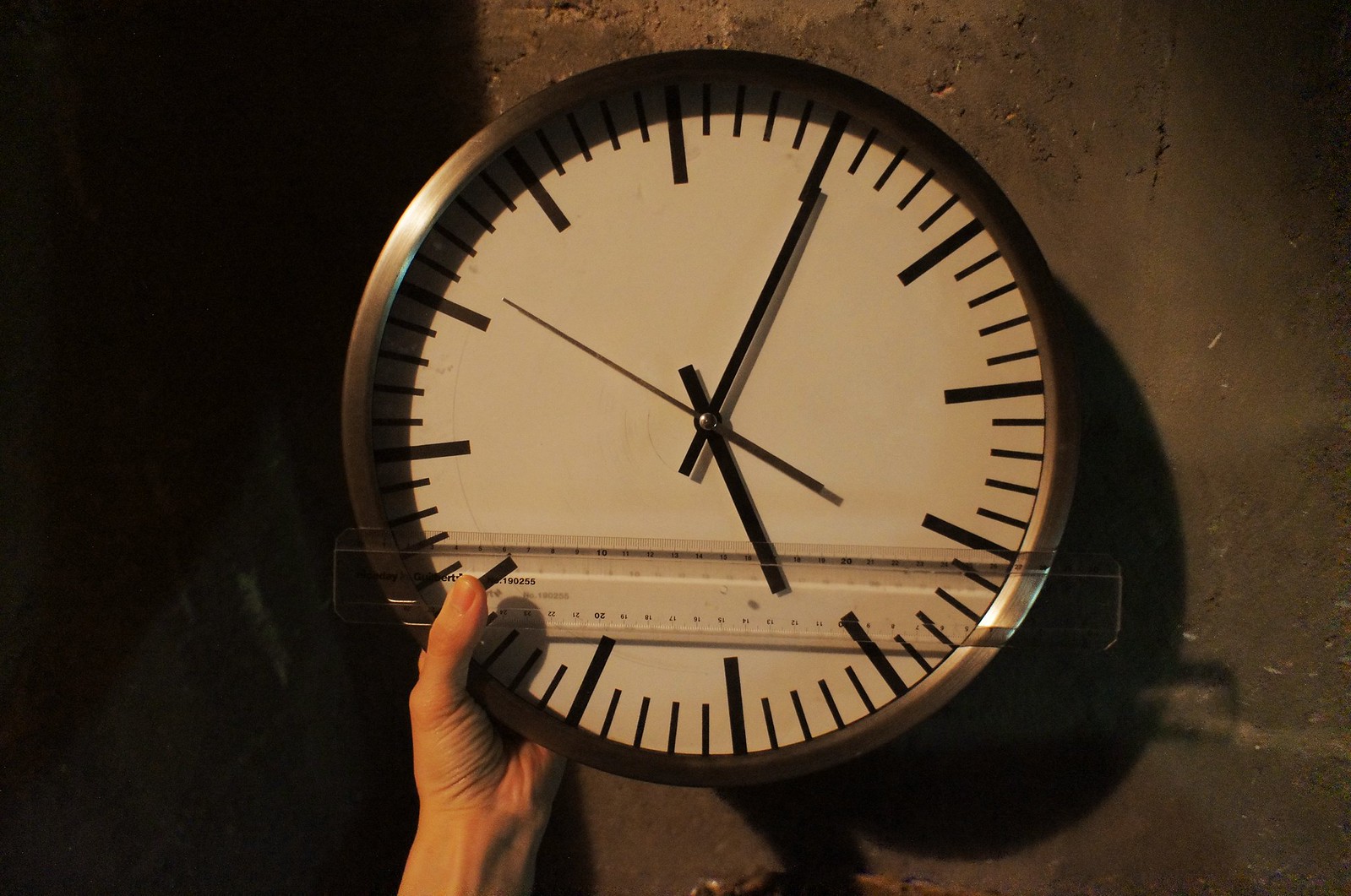A left hand is holding an analog clock against a cement wall. The clock is positioned in a well-lit area, while the left third of the image is cast in shadow. The hand holding the clock is outside the shaded area. The person's hand is also holding a clear ruler horizontally along the bottom edge of the clock to indicate its width. The clock features no numbers, only thicker lines to mark the hours and shorter lines for the minutes or seconds. The clock’s outer rim is copper-colored, while the face has a green hue. The clock hands and markings are black, and the orientation of the clock makes it difficult to discern the top or bottom.